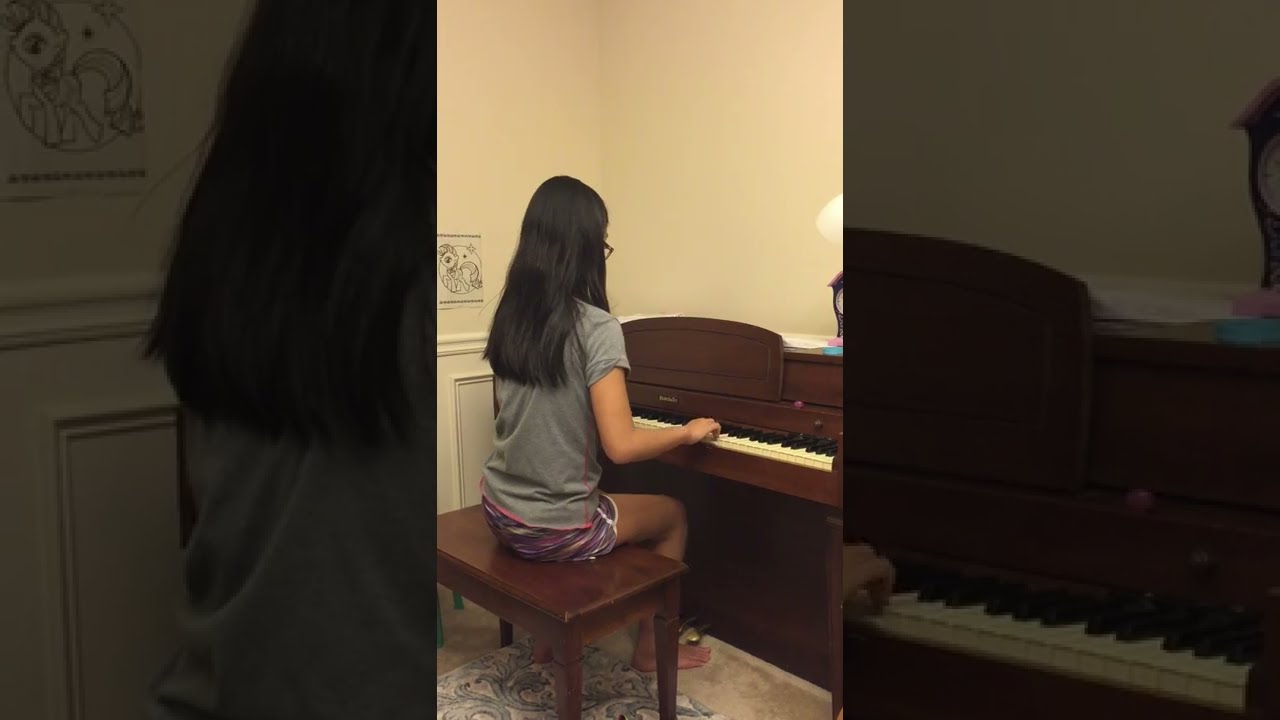In this detailed photograph, an Asian girl sits center-frame at a wooden piano, her back turned to the camera. She is dressed in a gray t-shirt and multicolored shorts that feature shades of purple, pink, and white. Her thick black hair, straight and lengthy, cascades down past her shoulders. Perched on a brown wooden bench, she leans forward slightly, focused intently on the piano keys, her hands poised over them as if playing from memory, since no music book is present.

The piano itself is a compact, old wooden model set against a yellow wall. At the bottom, gold pedals are just visible. A lamp rests on top of the piano, and to the left, partially obscured but discernible, is a piece of artwork or painting mounted on the wall. The child's eyewear includes black thick-framed glasses, though they're barely visible due to her angle. The setting appears to be an indoor space, possibly a bedroom or music room. The palette of the scene includes various colors like yellow, white, black, brown, purple, pink, gray, off-white, and green, providing a vibrant and welcoming atmosphere.